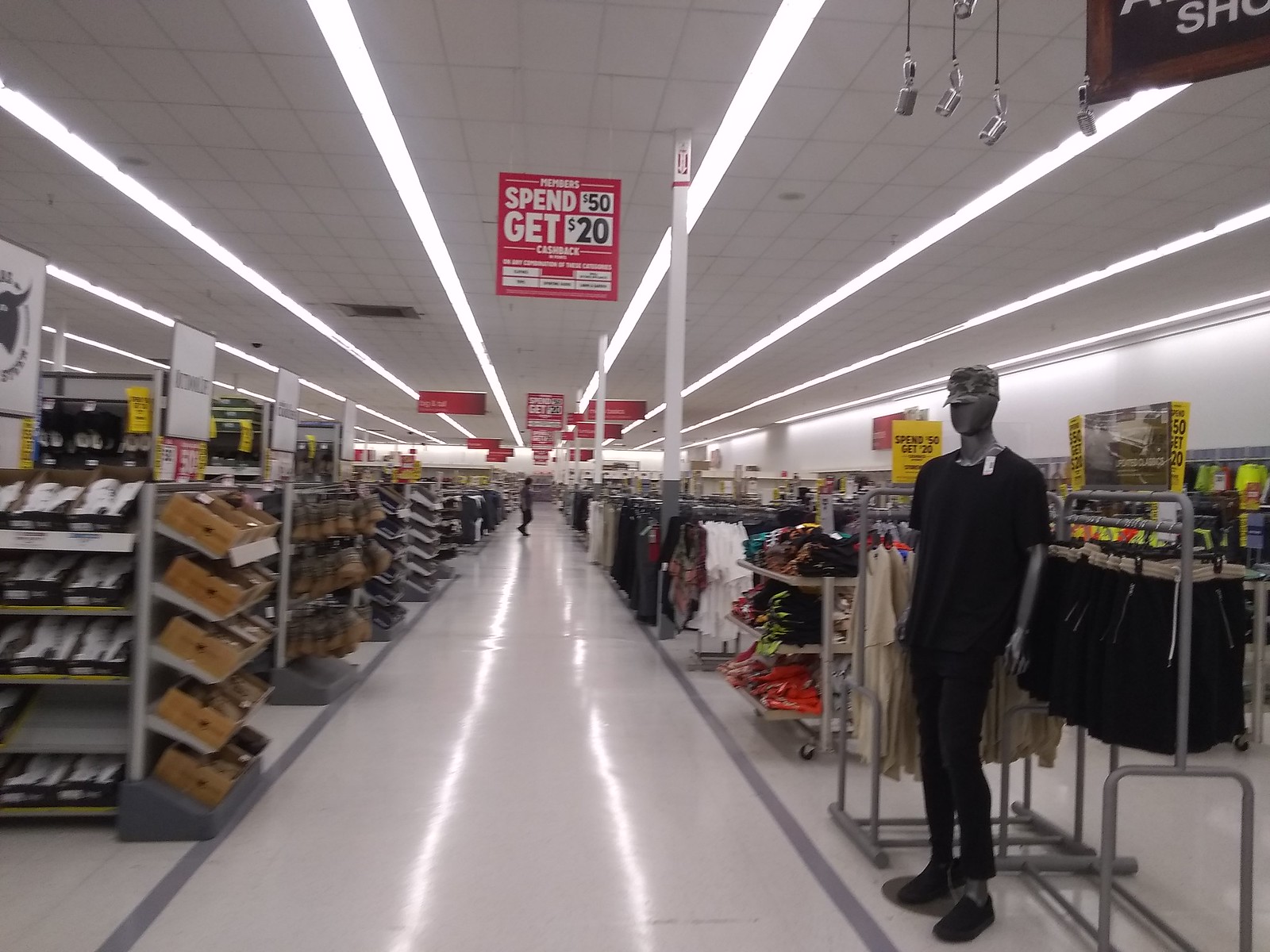The image is a color photograph taken indoors within a retail store that specializes in clothing and footwear. The viewer's perspective is down a central walkway, which extends far into the distance, lined with rails and racks filled with various articles of clothing and shoes. 

On the right side of the walkway stands a mannequin, dressed entirely in black, with a black top, trousers, and shoes. The ensemble is complemented by a camouflage baseball cap that features green tones, reminiscent of military headgear.

Suspended from the ceiling is a red sign prominently displaying a sale offer: "Spend $50, get $20 off." While additional text is present on the sign, it is too small to read from this vantage point. 

The scene is bathed in bright, uniform lighting provided by continuous strips of white lights affixed to the ceiling, ensuring the entire area is well-lit and inviting.